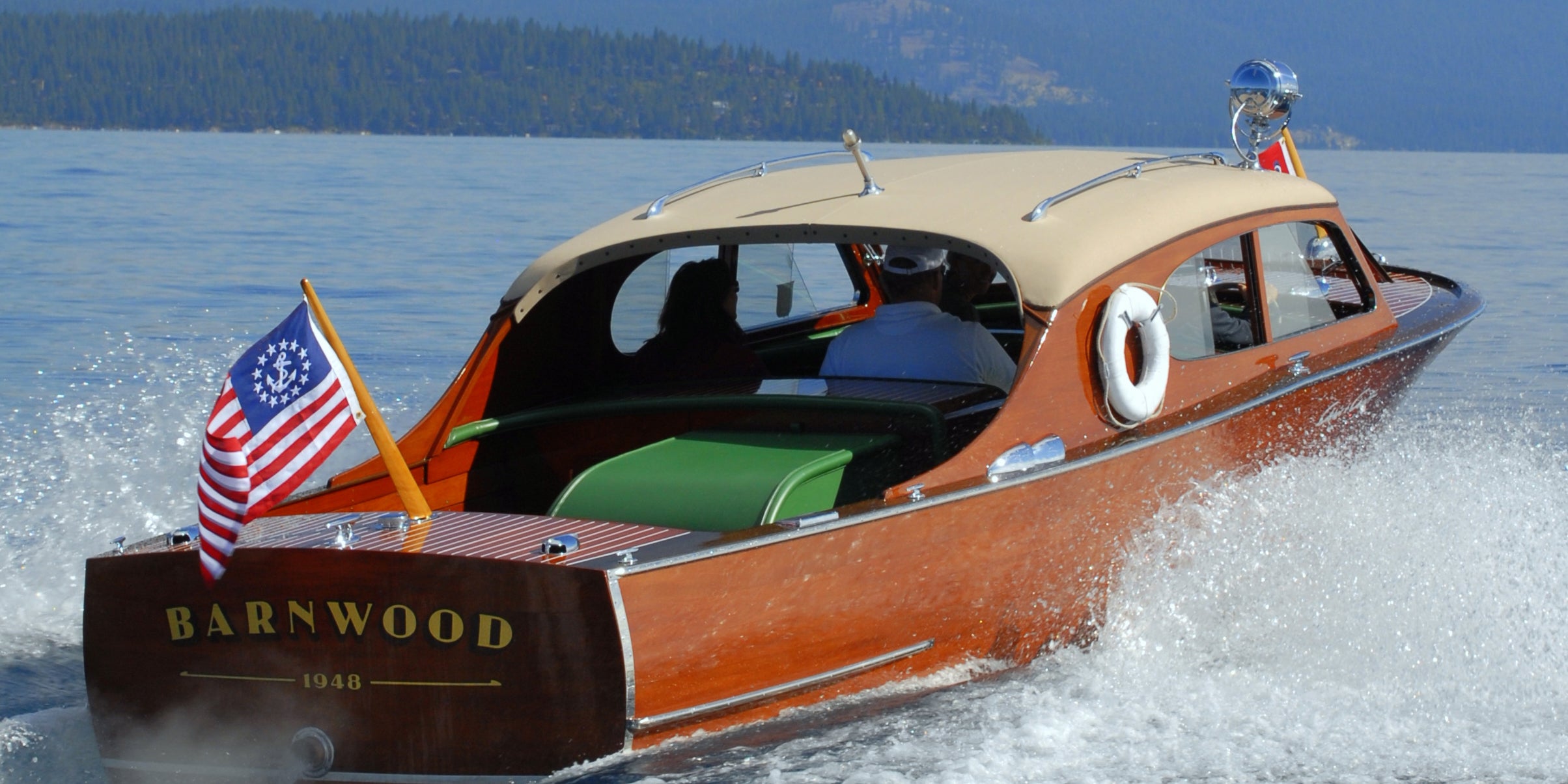The photograph captures a sleek, vintage speedboat from 1948 with a unique design that closely resembles a car. The boat is constructed from reddish-orange wood with brown panels, giving it a classic, old-fashioned appearance. The name "Barnwood 1948" is emblazoned in gold letters on the rear. The interior is accented with dark green details and features a large cabin with seating for at least four people. At the stern, an American flag, though slightly modified, flutters in the breeze, and a white life preserver is affixed to the side for safety. The vessel is actively racing through the water, creating lively splashes and ripples that emphasize its speed. Amidst this action, two passengers are clearly visible—a man and a woman—with the possibility of a third person silhouetted. The boat's stylish design includes elements such as a bright light signal at the front and numerous windows, blending the aesthetics of a car with the functionality of a boat. The background showcases a bright blue sky and a slightly out-of-focus forest, enhancing the scene's dynamic yet serene ambiance.